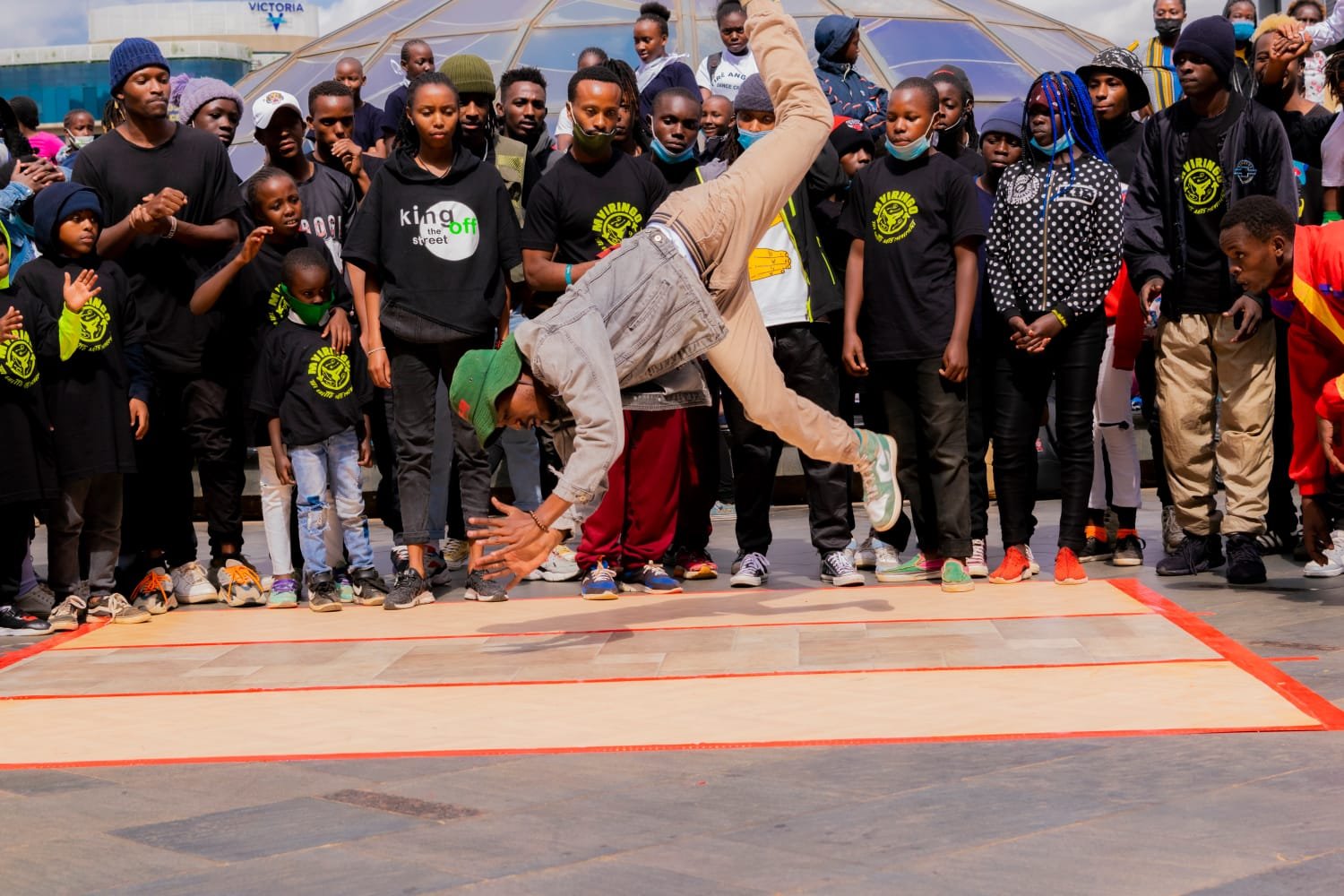The image captures a dynamic breakdancing performance by an African American male in mid-air, seemingly about to go upside down in a somersault. He is dressed in beige pants, a gray jacket, and a green hat. One leg is extended upward while the other is closer to the ground, with his head aimed downward and his hands reaching toward the floor, which is covered by a beige mat with orange edges placed on a gray concrete surface. A diverse crowd, predominantly African American and spanning various ages from children to young adults, closely observes the performance. Many in the audience wear COVID masks either under their chins or not at all. The background features a glass dome, providing a distinct setting to the scene. Among the spectators, a person with a gray and red jacket with a yellow stripe is noticeable on the right side of the image.